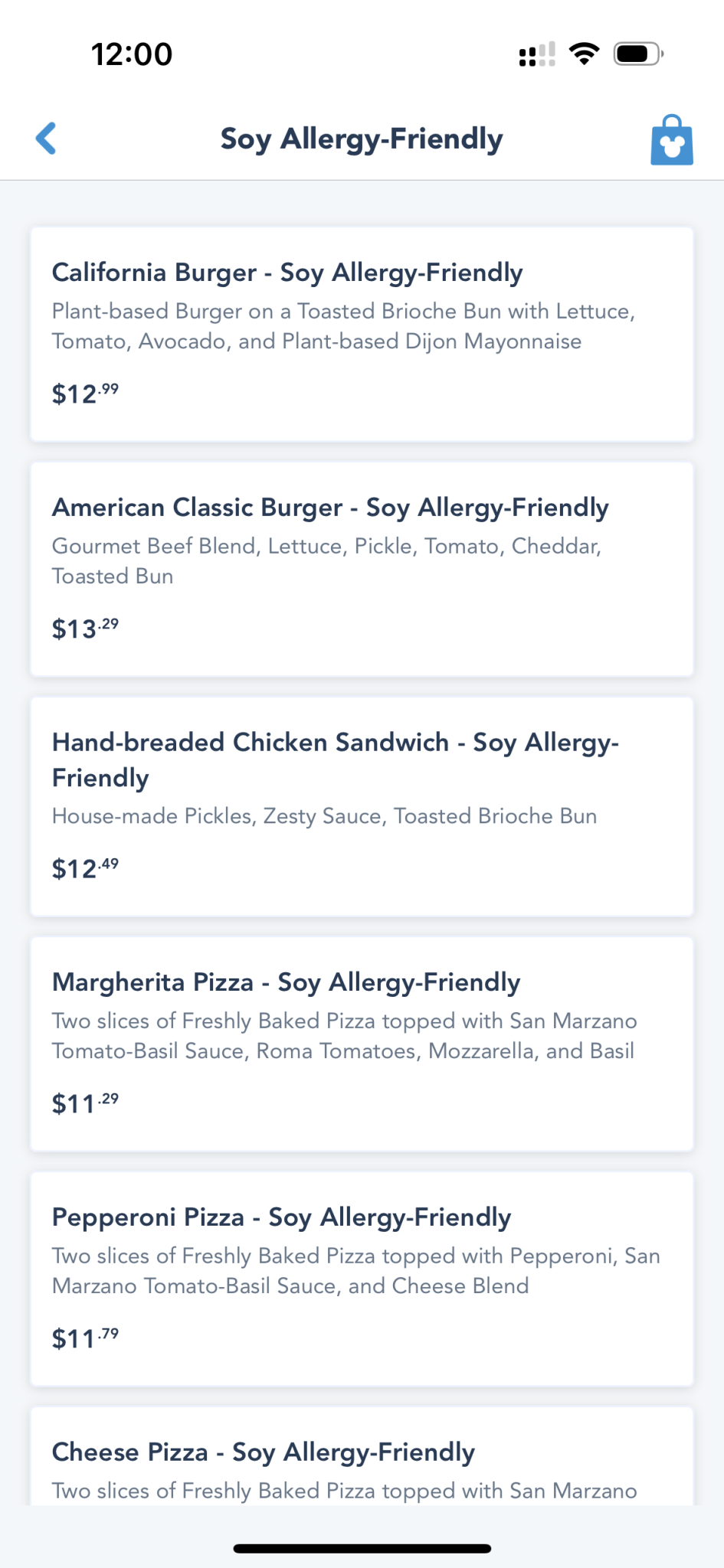In the top left corner of the image, the number "12" is displayed. Adjacent to it are two out of four bars indicating cellular signal strength, full bars representing Wi-Fi connectivity, and a battery symbol showing three-fourths charge. Below this, there is a back arrow and a shopping bag icon.

Featured in the image are the following soy allergy-friendly menu items:

1. **California Burger** - A plant-based burger served on a toasted brioche bun, garnished with fresh lettuce, tomato, avocado, and Dijon mayonnaise. Priced at $12.99.

2. **American Classic Burger** - A gourmet beef blend burger topped with lettuce, pickle, tomato, and cheddar cheese, served on a toasted bun. Priced at $13.99.

3. **Hand-Breaded Chicken Sandwich** - A sandwich consisting of crispy hand-breaded chicken, house-made pickles, and zesty sauce, all within a toasted brioche bun. Priced at $12.49.

4. **Margherita Pizza** - Two slices of freshly-baked pizza featuring San Marzano tomato basil sauce, Roma tomatoes, mozzarella, and basil. Priced at $11.29.

5. **Pepperoni Pizza** - Two slices of freshly-baked pizza topped with pepperoni, San Marzano tomato basil sauce, and a cheese blend. Priced at $11.79.

6. **Cheese Pizza** - Two slices of freshly-baked pizza topped with San Marzano tomato basil sauce and a cheese blend. Priced at $11.79.

The description cuts off with the word "black line," indicating possible text truncation.